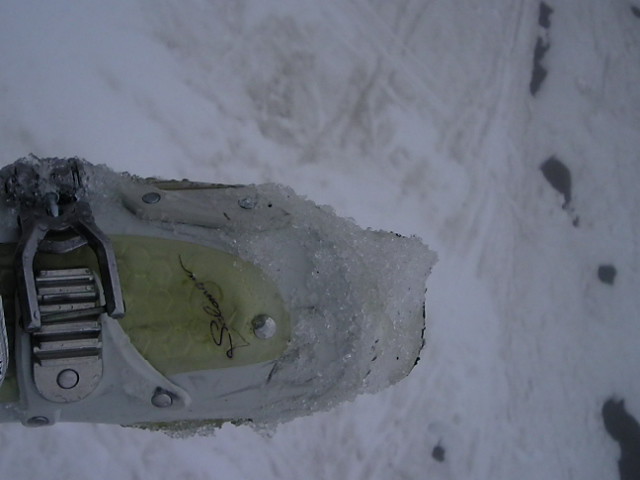The photograph captures the side view of a snowboarding or ski boot amidst a snowy backdrop. The boot spans from the left to the right of the image, with a distinctive gray metal or plastic buckle and several bolts and screws securing its structure. The boot's surface exhibits areas with white paint flaking off, revealing parts of yellowish-brown and metallic surfaces beneath. In the middle section of the boot, a cursive black signature is visible on a slightly ivory-toned patch. Surrounding the boot is a snowy ground, dirty with various brown, gray, and black blotches, as well as protruding black and brown rocks. There are scattered lines marking the snow's surface, giving it a textured and somewhat rugged appearance.